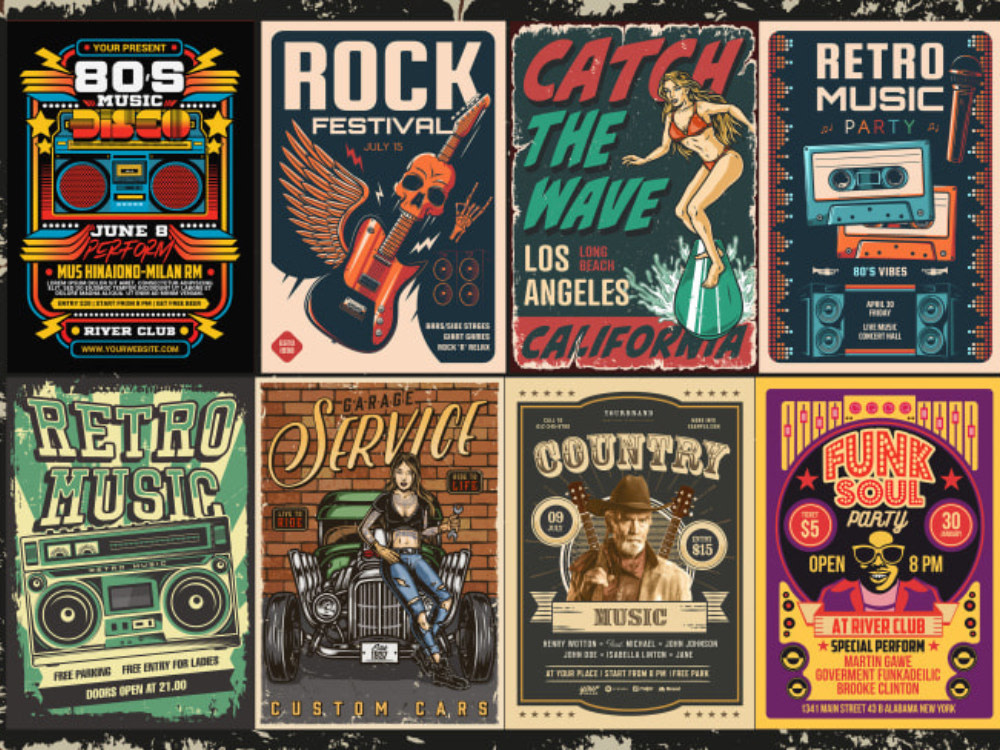This image features a series of eight classic retro music posters arranged in two rows of four against a black wall with white spots. Each poster offers a unique theme and vivid artwork. 

In the top row:
1. The first poster is an 80s-themed design with a retro blue stereo. It announces an event on June 8th at the River Club, highlighting the word "Perform" in red text, accompanied by smaller unreadable text and two cartoon lightning bolts.
2. Next is a Rock Festival poster featuring a striking electric guitar adorned with a skull and angel-like wing, with additional rock graphics like a skeletal hand throwing the rock sign and red cartoon lightning bolts. The white text on black and red diamond accents add to the festival's edgy feel.
3. Centrally placed is a vibrant 50s beach party poster that reads "Catch the Wave" in red and green. Beneath, it highlights Los Angeles and Long Beach, California, showcasing an illustration of a woman in a red bikini surfing on a green and white striped board.
4. The final poster in the top row captures the essence of a Retro Music Party. It includes a colorful mix of 80s vibes with illustrated cassette tapes and a boombox, and multicolored text stating "Party."

In the bottom row:
1. First is another retro-themed poster in green, black, and white, showing a boombox and the text "Retro Music" with smaller unreadable elements.
2. The next one is for Garage Service, displaying a stylish woman in ripped blue jeans and a small top, leaning against a retro green car adorned with various spoilers. Yellow text at the bottom states "Custom Cars," with additional license plate-like signs reading "Ride" and "Life."
3. The third poster advertises a Country Music concert, featuring a man in a cowboy hat with two guitar necks crossing behind him. The text is mostly in a stylized font, with noted details like a tan jacket and a red or brown bandana.
4. The final poster in the bottom row is for a Funk Soul Party, marked by a large afro-shaped illustration resembling a vinyl record. It promotes a performance on August 30th at the River Club for $5, and includes names like Martin Gaw, Government Funkadelic, and Brooke Clinton in small, readable text.

The shared elements of retro aesthetics and vibrant illustrations create a cohesive and nostalgic visual experience.